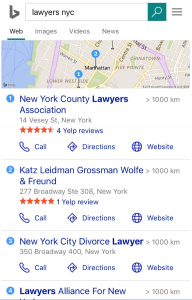A blurry screenshot of search results is depicted with a white background in the top left. An angular, lowercase, dark gray "b" is prominently displayed, where the top leg of the bulb does not connect to the stem. To the right, a white search box with a thin light gray outline shows black text that reads "lawyers NYC" in all lowercase letters. Next to the search box is a teal blue square featuring a white magnifying glass icon. Adjacent to this, outside the box, is a dark gray hamburger menu.

Below this, dark gray text reads "Web," underlined with a thick teal line. Nearby, in light gray text, are the options "Images," "Videos," and "News." Further down, a wide map image shows beige and green land with blue water on the left, crisscrossed by dashed dark blue lines. The land areas feature purple, pale yellow, and white roads in a grid-like arrangement.

The main body of the page has a white background and includes sections numbered 1 through 4 at the top left of each section. Each number is inside a bright blue circle with white numerals. To the right of the numbers, there is large blue text, followed by a light gray line of text indicating "carat pointing right, then 1,000 kilometers."